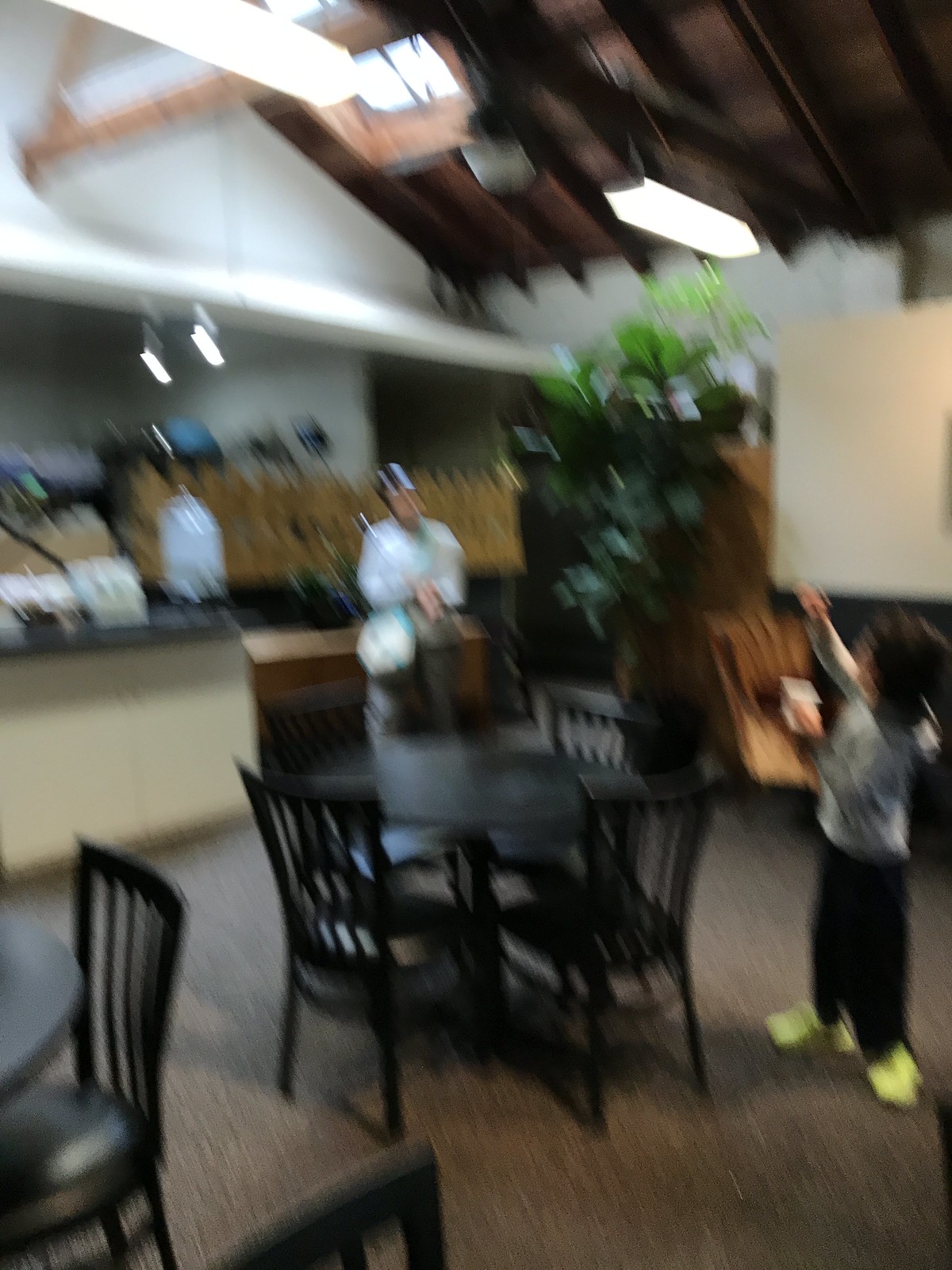This is a very detailed, but blurry photograph capturing the interior of a restaurant. The restaurant features white walls and a mix of dark brown and black furniture. Circular tables with matching chairs are prominently displayed, and the floor is a combination of tan and black speckles. In the center of the room, there is a large black flower pot with a lush green plant growing in it.

On the right side of the photo, a small boy, approximately six or seven years old, stands wearing yellow shoes, black pants, and a gray hoodie. He appears to be playing and has both hands up, possibly holding a cardboard sign, and has longish hair. In the background, there is a male chef seated behind what might be a counter or in the kitchen area, dressed in a white chef's jacket and gray pants. An interesting detail is that it looks like he has a pot on his head.

The ceiling of the restaurant is vaulted, with dark brown wooden beams contrasting against some white sections. A fluorescent white light fixture hangs from the ceiling, illuminating the space with a soft glow. Overall, despite the blur, the photo captures the cozy yet bustling atmosphere of the restaurant.